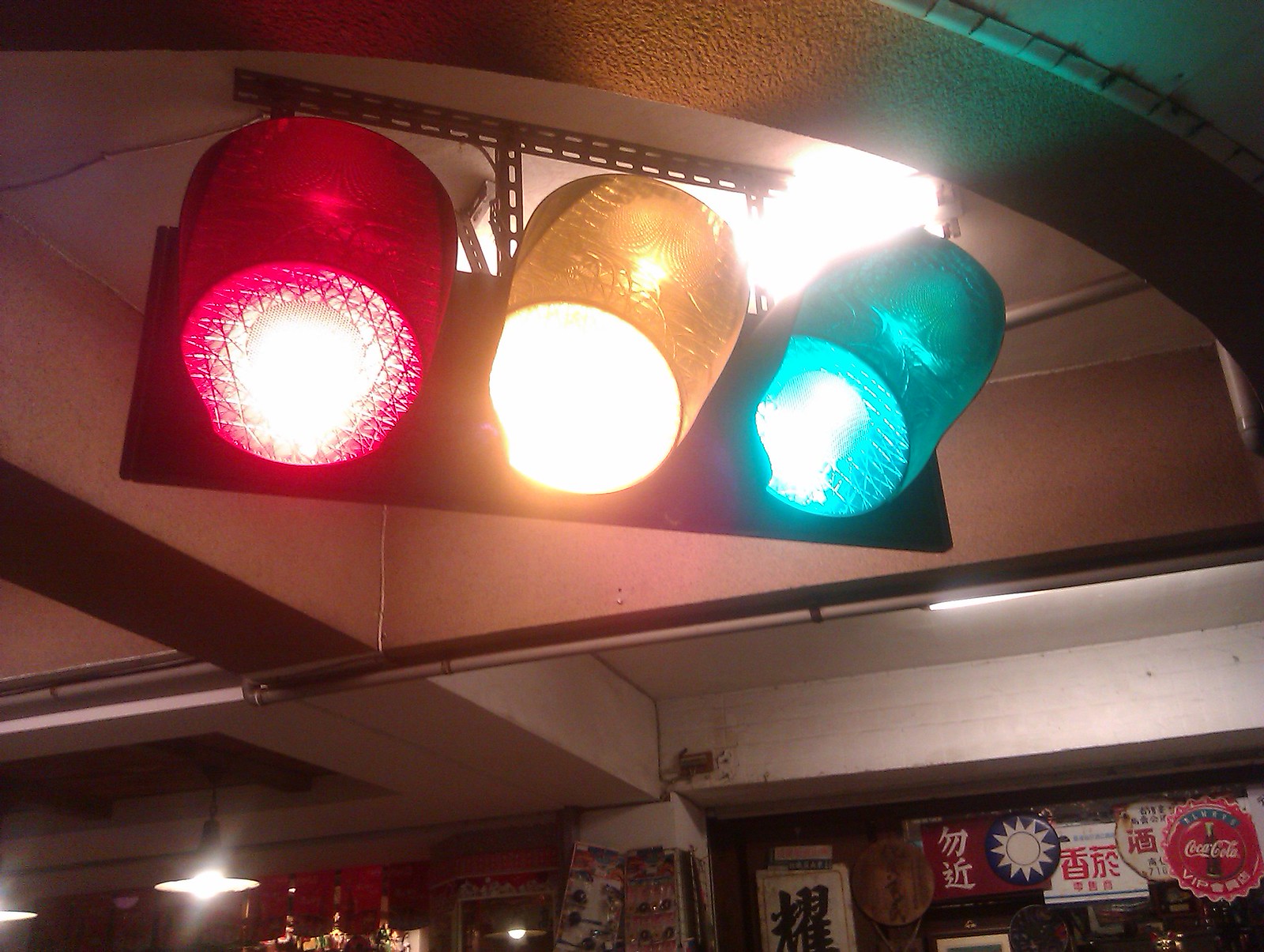The photograph captures an interior scene, most likely in a vibrant area resembling a Chinese alley, packed with shops and restaurants. The primary focus is on an atypical traffic light fixture hanging from a recessed cement ceiling with crossing beams. This artistic installation features three illuminated lights - a red bulb, a yellow bulb, and a green bulb - encased in sculpted, translucent glass. These colorful bulbs are arranged horizontally next to each other, and their unconventional placement and design lend an artistic feel to the space. The background is bustling with various logos, including a distinctive round Coca-Cola sign and numerous Chinese characters on plaques and posters. Additional hanging, shaded lamps contribute to the layered lighting. The scene hints at a lively, possibly bar-like environment with atmospheric elements that spark curiosity and intrigue.